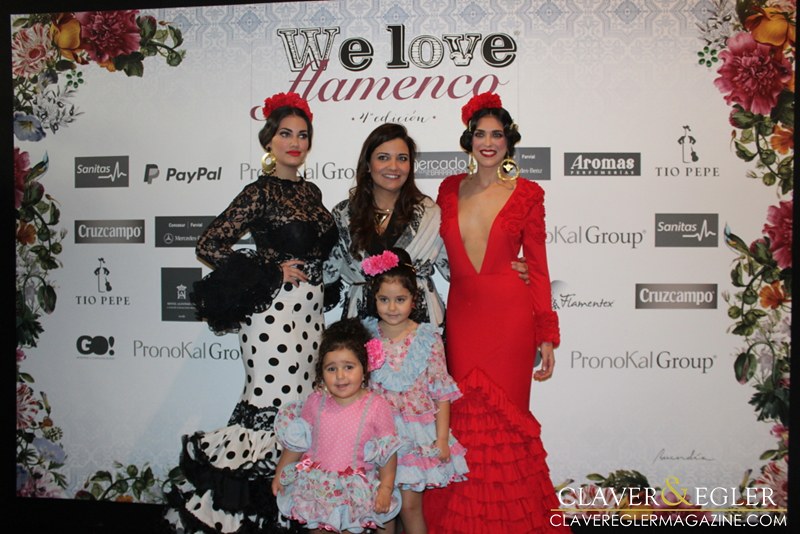This image, featured in CleverEgglerMagazine.com, showcases a vibrant flamenco-themed event prominently backed by numerous sponsors including Tio Pepe, PayPal, Aromas, Sanitas, Sinoxas, Prono Cow Group, Cruz Campo, Mercedes-Benz, and more. In the background, a decorated white curtain festooned with flowers prominently displays the phrase "We Love Flamenco," with "Flamenco" highlighted in bold red letters and "We Love" in white and black. 

Front and center are two young girls, approximately aged two and four, dressed in endearing pink and white fluffy flamenco attire with pink accents in their hair, indicating their budding interest in flamenco dancing. Surrounding them are three elegantly dressed women in vibrant flamenco outfits. The woman on the left dazzles in a long polka dot dress, a black latticed blouse with wide sleeves, a striking red hair accessory, and statement gold earrings. The central figure drapes a white robe over her shoulders, adorned with a gold necklace, and her long brown hair flowing gracefully. The woman on the right commands attention in a deep v-neck red dress reaching her navel, complemented by a red hat, black hair, and golden earrings.

This lively snapshot also includes the presence of the magazine's editor or owner, seen standing next to the flamenco dancers, further emblematic of the support and celebration of flamenco culture championed by Clever and Eggler Magazine.